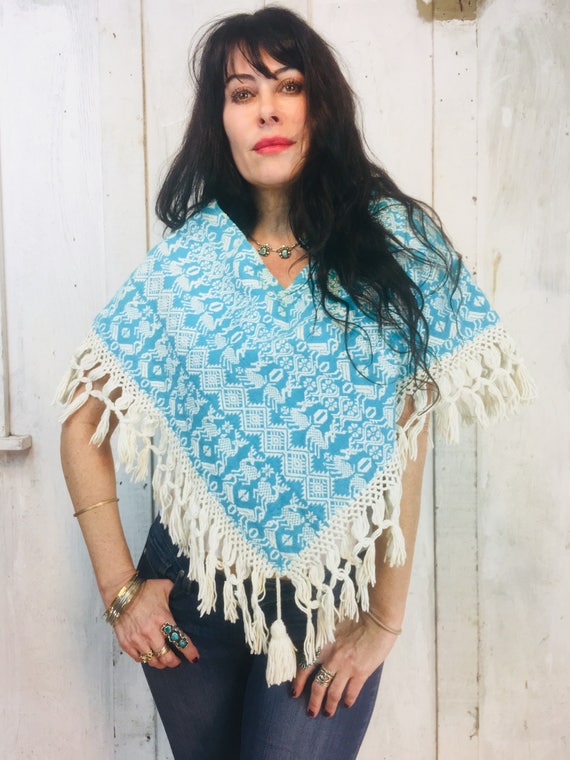In this photograph, a woman stands gracefully centered against a white or light gray painted wood wall, which has some areas of gray. She has long, slightly wavy black hair, which is pulled back on her right side and cascades over her left shoulder. Sporting a red lipstick and detailed eye makeup, including mascara, black eyeliner, and brown eyeshadow, her complexion appears very pale. She also has bangs and black eyebrows framing her brown eyes. She is adorned with a turquoise necklace. 

She wears a striking blue and white shawl-like poncho, featuring intricate white designs against the blue fabric and edged with white tassels that cascade around the garment. This attire creates a V at the waist and a modest V-neck at the top. Her outfit is completed with blue jeans, and she is posed with her right thumb in her right pocket, her hand resting on her hip, and her left hand on her left hip.

Her accessories are a showcase of mixed metals: a turquoise ring on her right forefinger, two gold rings, two silver rings, a gold bracelet, and another bracelet on her right forearm, along with a bracelet on her left wrist and a ring on her left middle finger. The photograph cuts off just above her knees, giving a partial view of her outfit and pose.